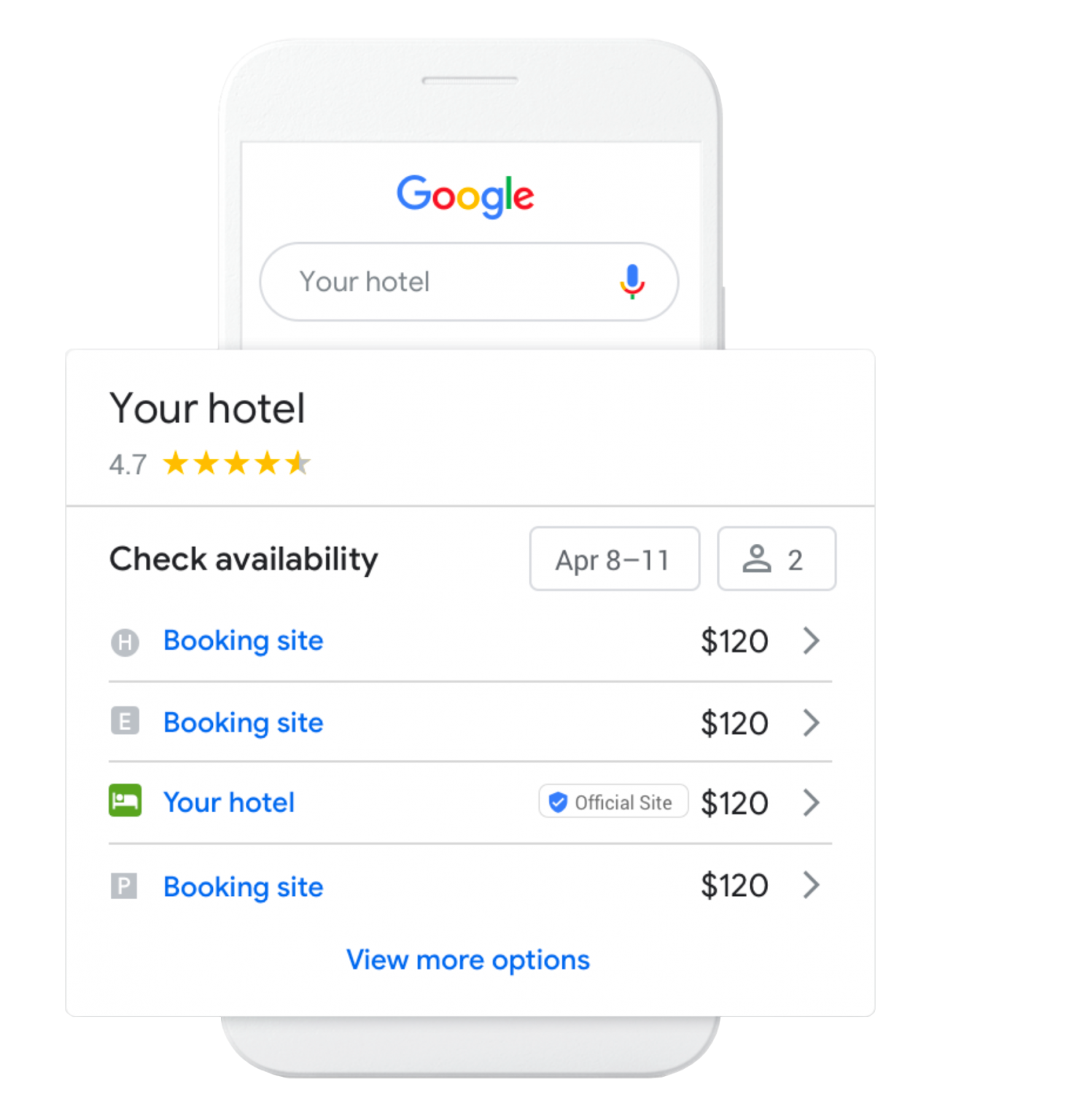Screenshot of a hotel listing with a 4.7-star rating, comparing prices between the official website and a booking site. The cost for a stay from April 8th to 11th for two people is approximately $120. The backdrop shows a Google search interface, with "booking site" highlighted in blue text.